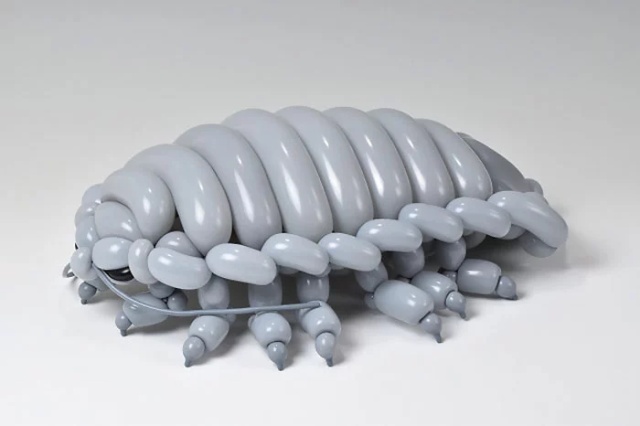The black-and-white image features an intricately crafted balloon animal designed to resemble an insect, possibly a beetle, due to its eight legs – six on the side and two front legs. The creature is positioned broadside and faces left. The body structure comprises long, tubular balloons forming an armadillo-like shell, accented by smaller, jelly bean-sized balloons lining the sides. Each leg ends in a sharp, claw-like point. An eye, characterized by a horizontal black slit, is centrally located on the side of its head. The background of the image is a dull gray, enhancing the detailed craftsmanship of the balloon creation.